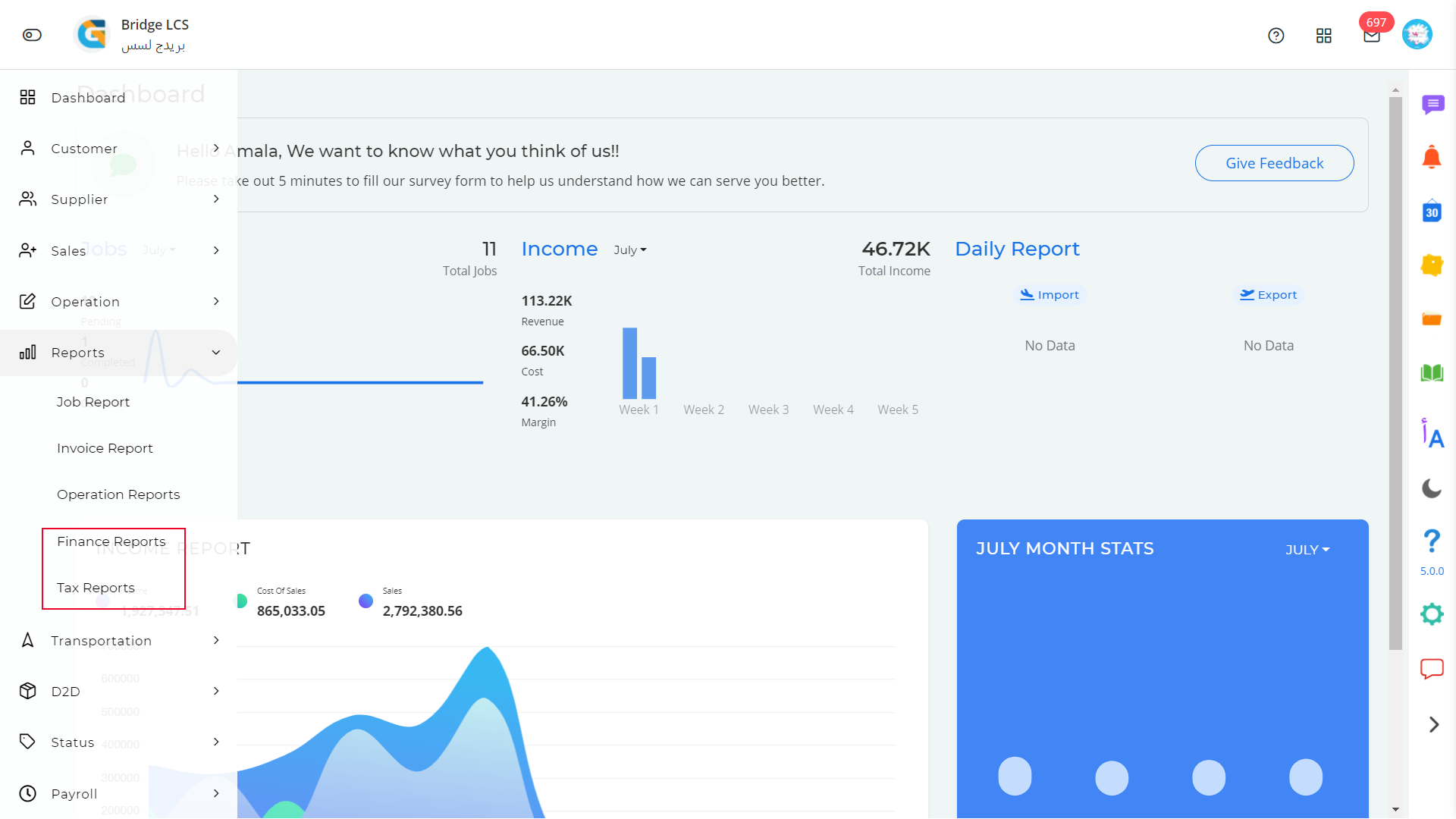The image depicts a website interface that currently lacks a visible name. In the top left corner, there is a profile icon labeled "Bridge LCS". Moving to the top right corner, a notification or email icon displays the number 697 against a red background. Adjacent to it is a light blue circle with a white icon in the center.

On the left-hand side of the screen, a vertical menu lists categories in the following order: Dashboard, Customer, Supplier, Sales, Operation, and Reports. Under the Reports category, subcategories are highlighted, with red squares emphasizing "Finance Reports" and "Tax Reports". Below these are further categories: Transportation, possibly denoted as "T2D", followed by Status, and finally Payroll.

The right upper half of the screen features a light gray background containing a chart and various data elements such as income and daily reports. At the top left of this section, a blue oval-shaped button labeled "Get Feedback" is visible. 

Below the light gray section, a chart with curvy lines rests on a white background. Adjacent to this on the right is a section titled "July Month Stats" highlighted with a blue square. At the bottom of this part of the screen, there are four white circles lined up to complete the interface.